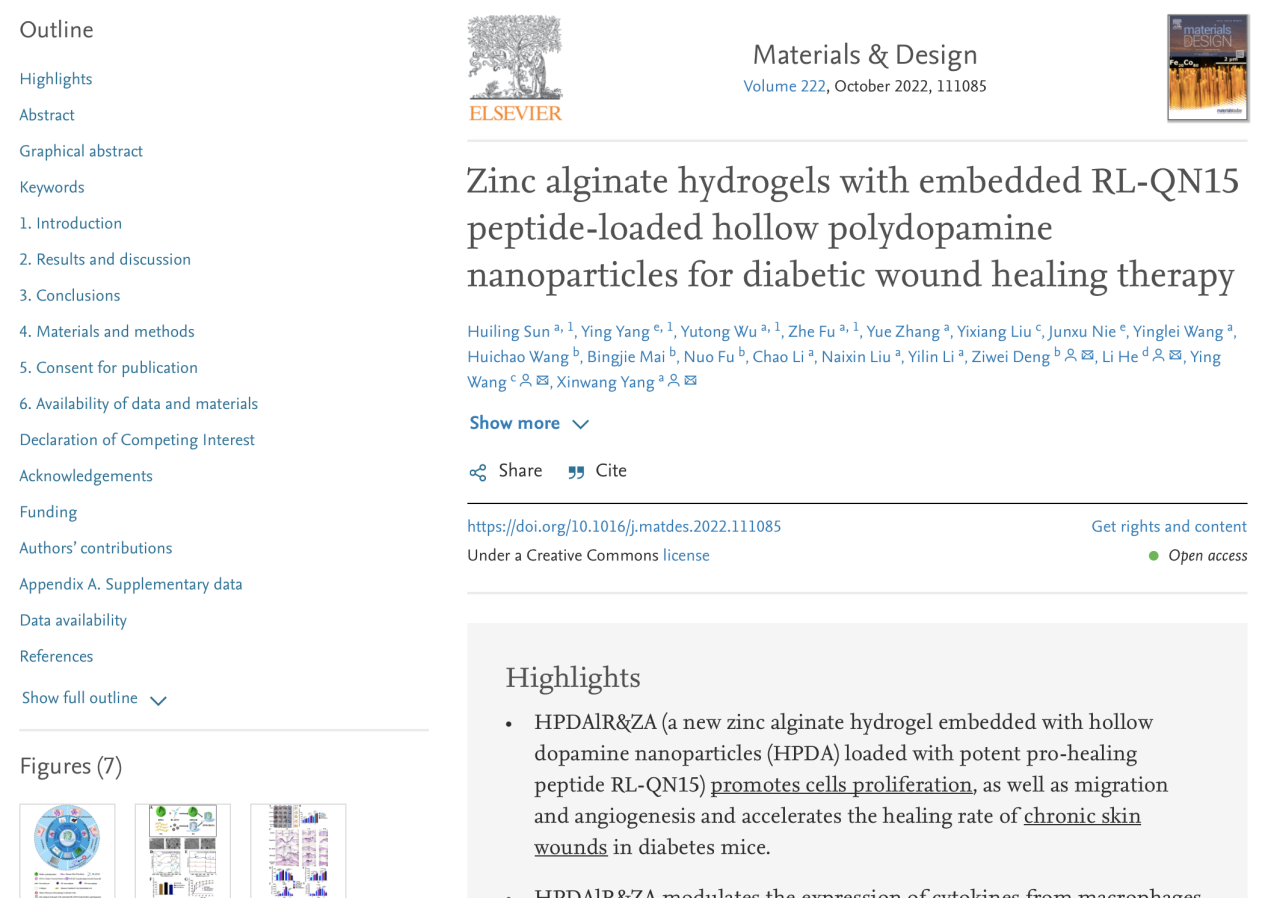In this image, the background is predominantly white with various text and elements arranged throughout. 

On the left side, a blue side menu is visible, with the top label reading "Outline." The sidebar contains an organized list of sections, including: 
- Highlights
- Abstract
- Graphical Abstract
- Keywords
- 1. Introduction
- 2. Results and Discussion
- 3. Conclusion
- 4. Materials and Methods
- 5. Consents for Publication
- 6. Availability of Data and Materials
- Declaration of Competing Interest
- Acknowledgements
- Funding
- Outcomes
- Contributions
- Appendix A
- Supplementary Data
- Data Availability
- References
- Show
- Food
- Outline

At the bottom of this sidebar, the label "Figure 7" appears, although three figures are actually presented on the bottom left corner of the page.

On the main page, a logo featuring a grey tree with the word "Elsevier" in orange beneath it is positioned in the top left corner. Centrally at the top, the title "Materials and Design, Volume 222, October 22, 11, 1085" is displayed in black text, with a book icon to its right.

Below these details, the main title reads "Zinc Alginate Hydrogels with Embedded RLQN15 Peptide Loaded Halopolydopamine Nanoparticles for Diabetic Wound Healing Therapy." This text is followed by the authors' names, written in blue and various languages.

A blue "show more" dropdown feature is available, followed by a URL, "doi.org." Additionally, a section labeled "Highlights" lists key points about the research:
- HPDALRNZA: New Zinc-Alginate Hydrogel Embedded with Halopolydopamine Nanoparticles (HPDA), Loaded with Wheat Peptide Pro-Healing Peptide RLQN15.
- Promotes Cell Purification, Migration, and Angiogenesis.
- Accelerates Healing Rate of Chronic Skin Wounds in Diabetic Mice.